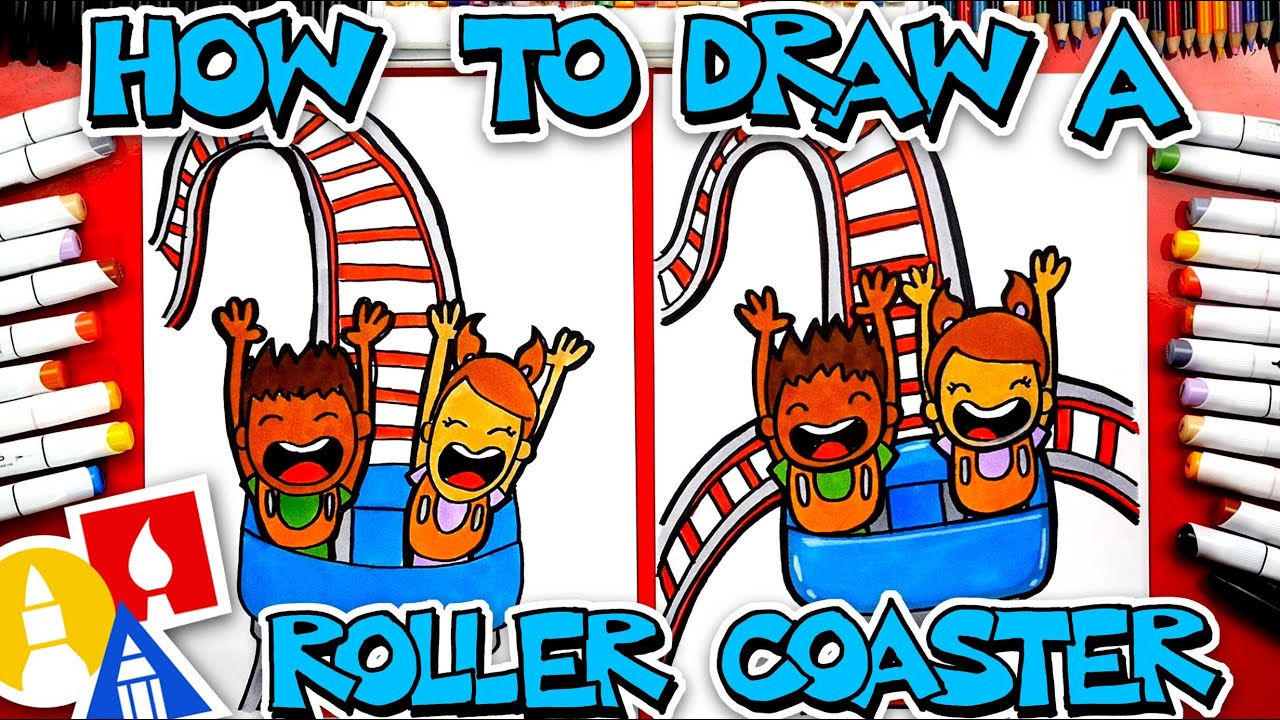The image features a step-by-step guide titled "How to Draw a Roller Coaster," displayed in turquoise letters outlined in black and white. The scene is horizontally oriented and showcases two illustrated roller coaster scenes, each slightly different, as though drawn by different people. Both illustrations depict a cheerful moment with two children, a brown-skinned boy with bushy hair and a lighter-skinned girl with red pigtails, riding a blue roller coaster cart. The kids have their hands raised enthusiastically, simulating the thrill of coming off a loop. The roller coaster tracks are distinctively red and white, with the right-hand drawing including additional intersecting horizontal tracks not present in the left-hand image. Surrounding both sides of the picture are colored pencils or artist's crayons, emphasizing the drawing theme. The children’s mouths are open in excitement, bringing a lively, animated feel to the instructional guide.